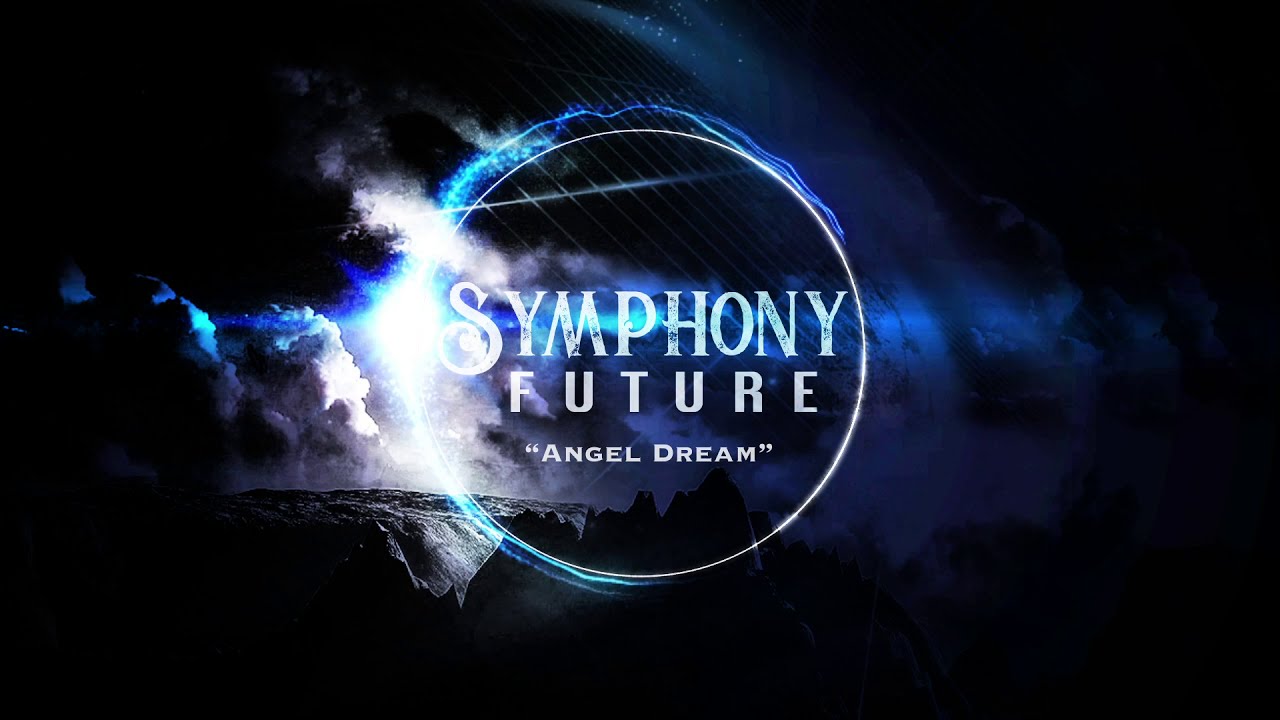The digital artwork, titled "Angel Dream" by Symphony Future, serves as a dramatic and visually striking advertisement. The image features a predominantly dark background interspersed with hues of blue and purple. Central to the composition is a thin-lined white circle, bordered by an electric blue aura reminiscent of an eclipsed sun. This central circle is set against a backdrop of heavy, gray and white storm clouds, jagged black mountains, and perhaps a waterfall. Sun rays break through an opening in the clouds, casting light amidst the dark scene. The image also incorporates elements that look like lightning or electric currents surrounding the circle's edge. Written in a mix of white and blue lettering, the names "Symphony Future" and "Angel Dream" are prominently displayed. Above the composition, a star field appears to cast its glow through a bright spotlight, further enhancing the surreal and dramatic atmosphere. The artwork suggests the symphonic and dramatic nature of Symphony Future's music, specifically their piece titled "Angel Dream."